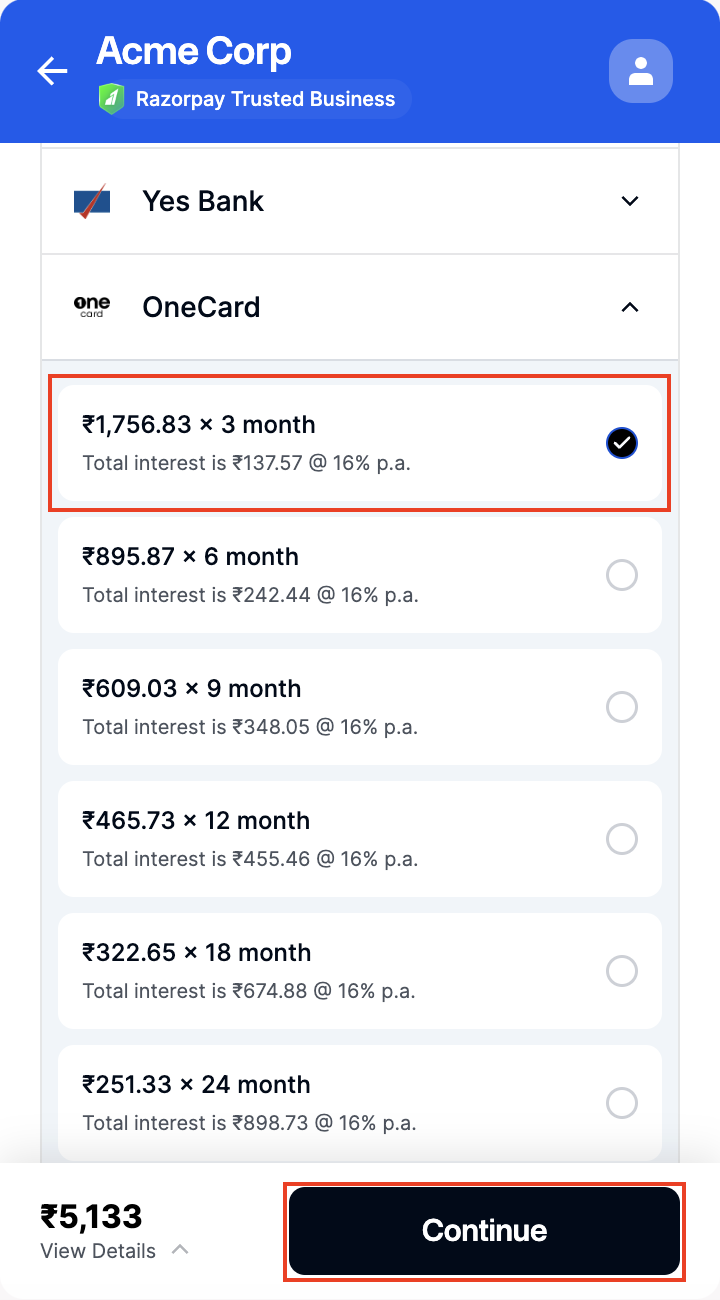In the center of the image is the logo of Acme Corp. To the left of the logo, there's a blue square with a light blue outline containing the letter "A", and to the left of that is a left-facing arrow. Directly below the Acme Corp logo, the phrases "Razor Play" and "Trusted Business" are displayed.

To the right of the logo, there is an "X" followed by a dropdown menu featuring an "A" inside a square. Below this, set against a white background, there is text that is partially cut off, reading "From 294 rupee/month" along with another dropdown menu.

A grey line separates this section from the next, which lists various banks along with their introductory offers. It begins with "Bank of Baroda, B-A-R-O-D-A," offering services starting "From 294 rupee/month" with an associated dropdown menu. Following this is "Federal Bank," with an offer of "From 291 rupee/month" alongside another dropdown option.

Outlined in blue is the next section, labeled "One Card". It includes various details such as a monthly cost of "2053.56 rupees" over a period of three months, a total interest of "160.80 rupees" at an annual rate of 16%, and a blue circle featuring a white check mark.

Concluding the image is a grey line with the phrase "Full amount of."